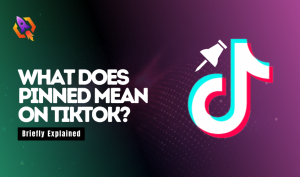The image features a horizontally elongated rectangle. The background transitions smoothly from bright green on the left to dark purple on the right, becoming darker green in between. Towards the right side, the purple shade lightens progressively into a brighter purple.

In the upper left corner, there is a striking hexagon that is yellow and orange. At its center, a purple rocket, with gradients of lighter purple, streaks through the hexagon. The rocket is depicted with vibrant flames at the bottom in shades of red and yellow.

Below this hexagon, bold white text reads: "WHAT DOES PINNED MEAN ON TIKTOK?" The large, capitalized font ensures the question stands out. Beneath this text, there is a prominent black button with the words "Briefly Explained" written in white font.

Adjacent to the text, the TikTok logo is depicted in white with a distinctive red drop shadow below and a turquoise shadow above. Accompanying the logo is a white pin icon positioned above it.

The color palette of the image includes hues of turquoise, red, purple, green, orange, yellow, white, and black. Additionally, the purple segment of the background features a pattern of dots, adding texture to the design.